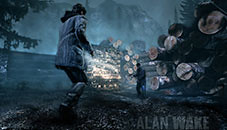A small, rectangular image appears to depict a scene from a computer video game. In the foreground, a man dressed in distinctive attire seems to be engaged in combat with an indistinct, white figure. The scene is set outdoors under a dark, bluish-tinted sky. The background features various objects, including barrels, contributing to the immersive environment. At the bottom of the image, a watermark bears the name "Alan Wake," suggesting a connection to the game's creator or main character.